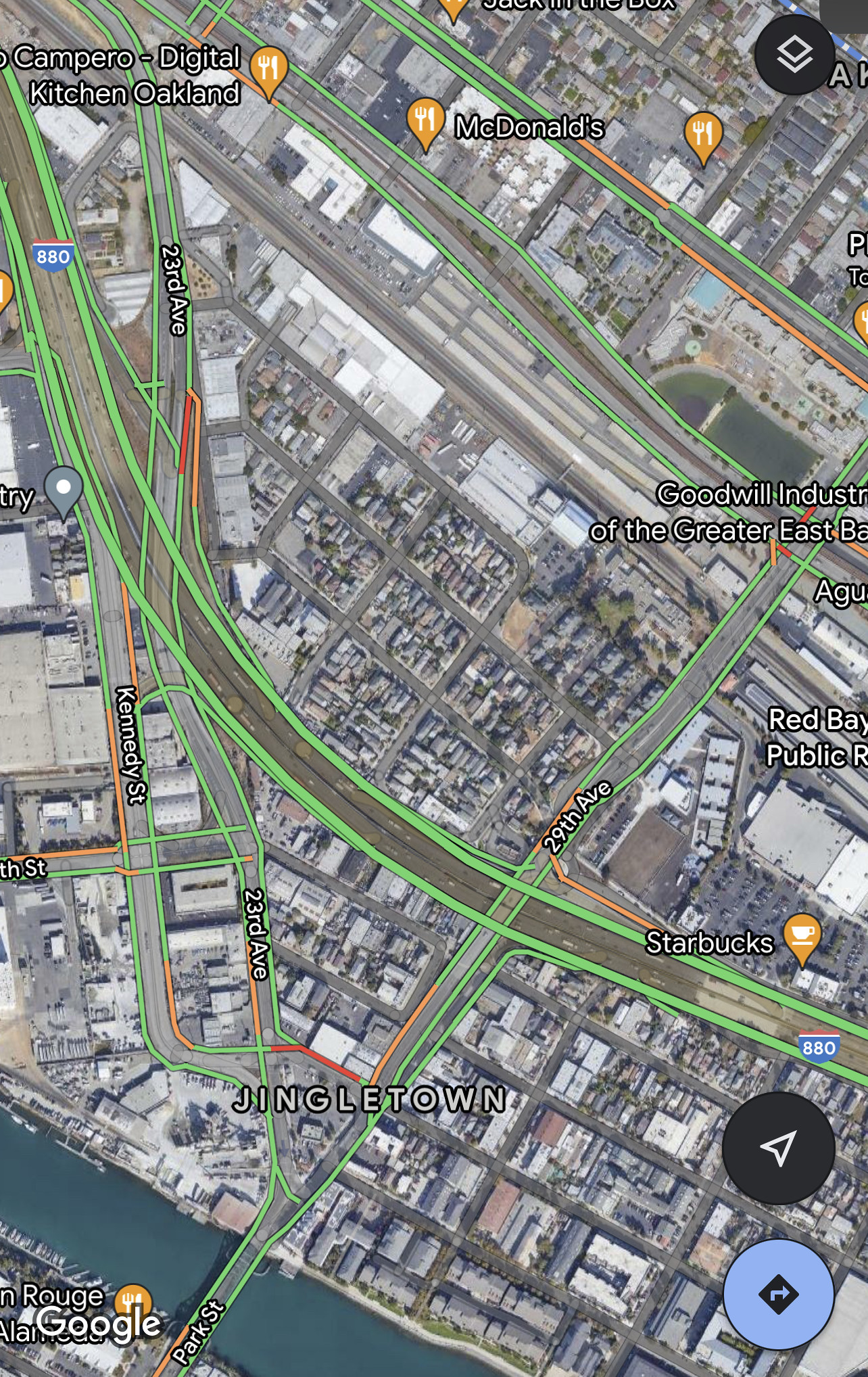This satellite GPS map image presents a detailed view of an urban area with distinct real-life colors depicting streets and buildings. Overlaid on the satellite imagery are GPS lines, highlighting streets in green, moderate traffic in orange, and heavy traffic in red. Various landmarks and street names are discernible:

- "Goodwill Industries of the Greater East B.A."
- "Red Bay Public (incomplete text)"
- 29th Avenue
- Kennedy Street
- 23rd Avenue (appears twice)

Prominent establishments in the vicinity include:
- Starbucks (two locations)
- McDonald's
- Comparo Digital Kitchen Oakland

The focal point of the map image is the intersection of Highway 880 (Interstate 880) and 29th Avenue, in the area known as Jingle Town, near one of the Starbucks locations.